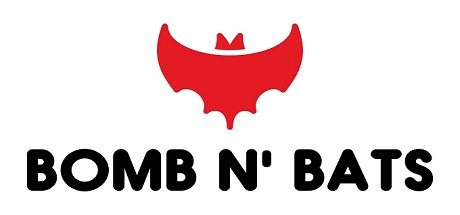The image is a computer-generated logo against a completely white background. Centrally positioned at the top is an abstract, red bat symbol composed of triangular shapes representing the ears, and rounded wings with notched edges that resemble bat wings. Above the bat's head is a small crown-like element. Below the bat, in bold, black, all-capital letters, the text "BOM & BATS" is displayed in rounded, blocky font. The overall design suggests it's a logo, possibly for a product, company, or advertisement, though its exact purpose isn't clear.